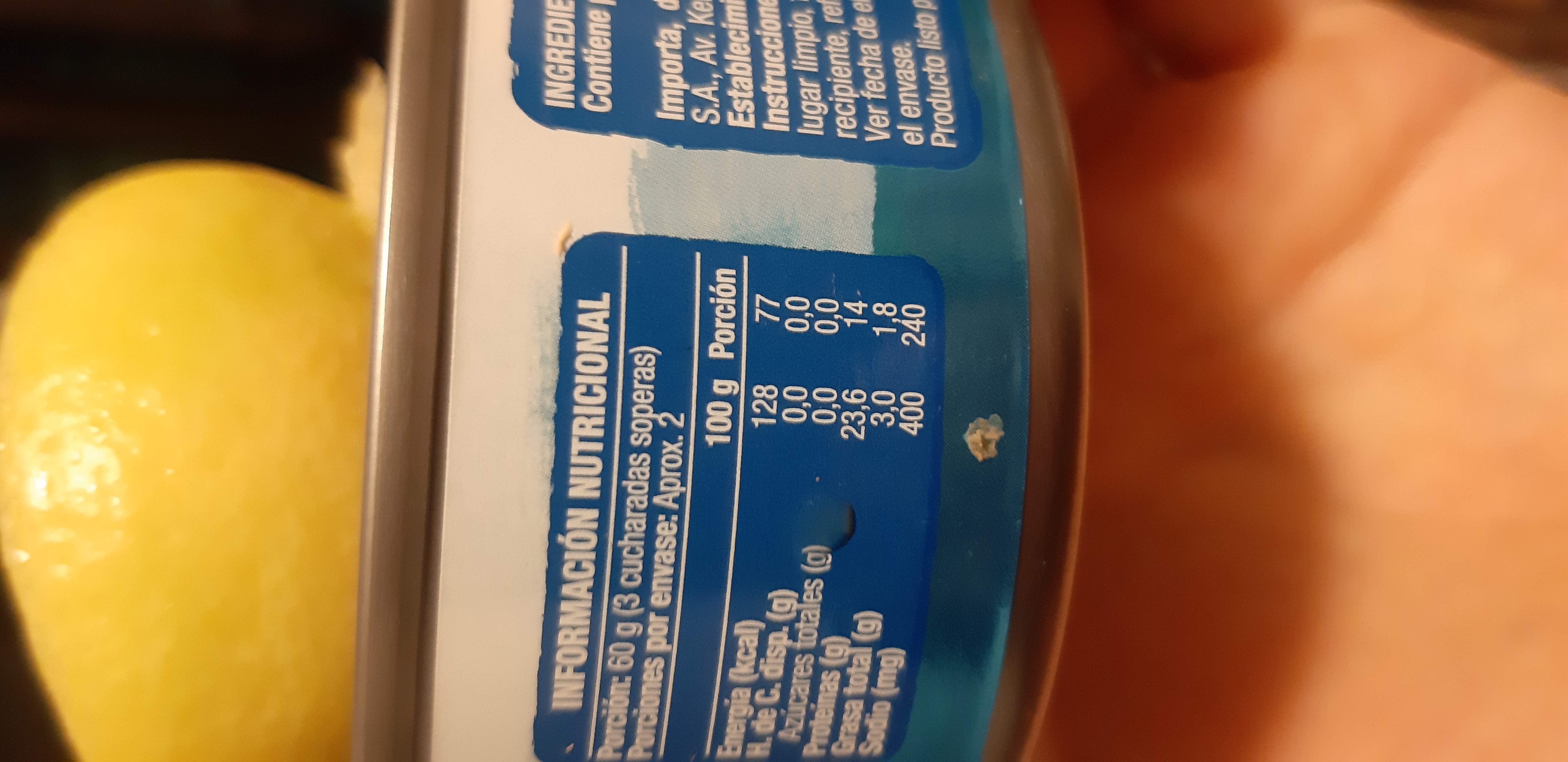This image is a horizontally-oriented color close-up photograph of a can, likely containing tuna, held in a hand with the palm facing upwards. The can, originally horizontal, appears vertical due to the image being tilted 90 degrees to the left. The can is predominantly white and aqua blue with a silver rim. It features two blue labels with white text, one displaying nutritional information and the other listing ingredients, both in a foreign language, possibly Spanish. To the left of the can, there's a bright yellow object that resembles a lemon, and part of a palm is visible, though blurred. The background is black, making the can and lemon stand out prominently.